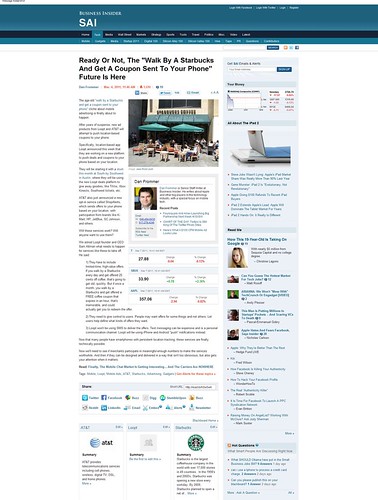The image features a promotional poster with a teal-colored section covering part of the upper half. Within this section, black text is present, but it's difficult to make out due to the zoom level. The upper left-hand corner above the border is not clearly visible, and even large white words within the border are hard to decipher. Prominently displayed in large letters is "S-A-I". Below this section, the background transitions to black. The title reads, "Ready or not, to walk by a Starbucks and get a coupon sent to your phone. Future is here." The author of the text is obscured, with only some indiscernible red and black text visible.

The outdoor setting includes a recognizable Starbucks location, marked by two teal-colored umbrellas where people are seated. The individuals appear blurry, and their specific features are not clear, though beige chairs are visible. In the middle of the image, there is a gray outline of a man wearing a white collared shirt and a black blazer; his other features are not distinguishable due to the blurriness. Towards the bottom, the AT&T logo is clearly shown along with a green, black, and white Starbucks logo.